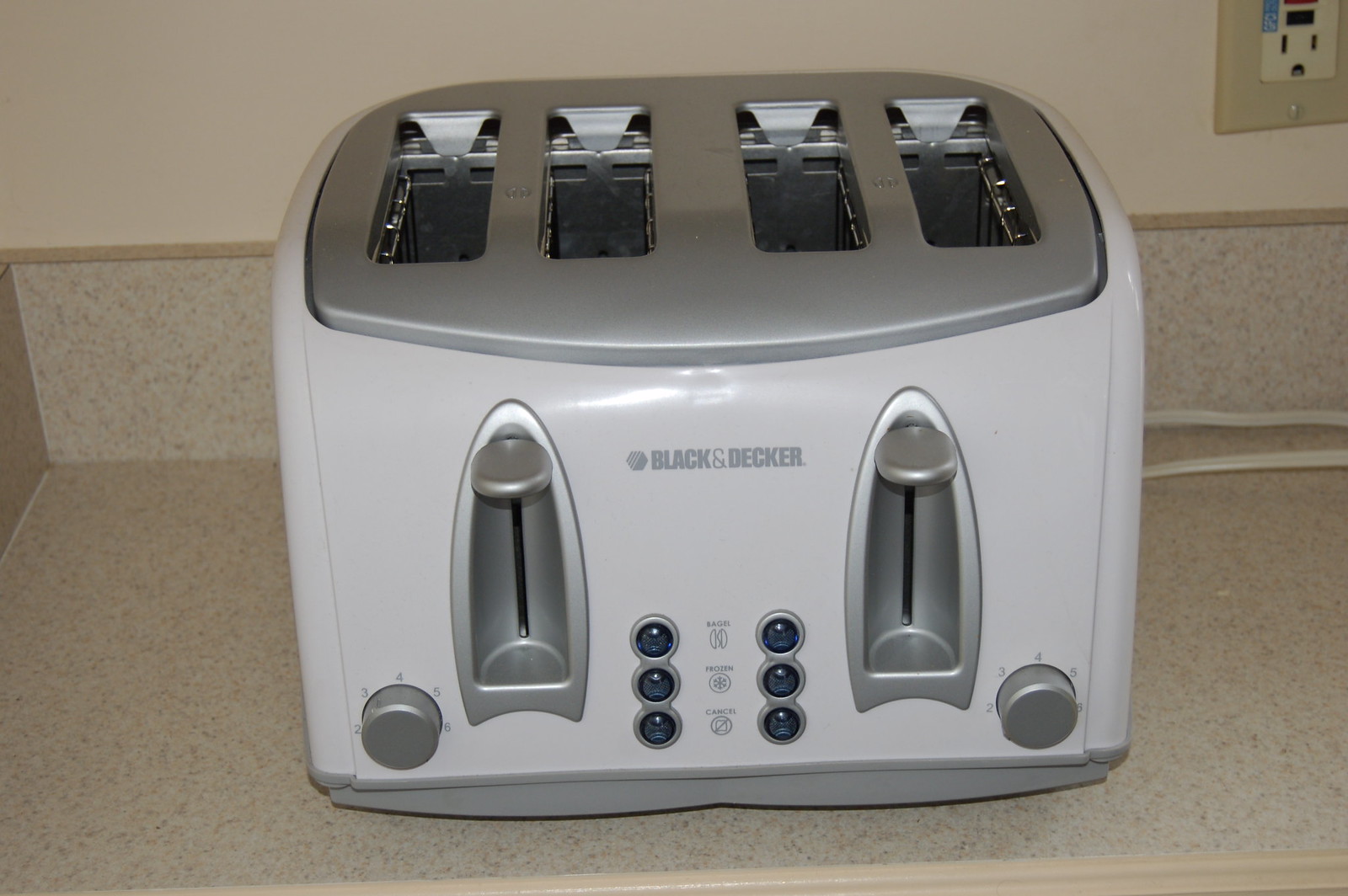This image depicts a Black & Decker toaster sitting on a patterned, cream-white kitchen countertop with a darker beige backsplash. The toaster, predominantly white with a silver top, has four slots for bread. The front displays the Black & Decker logo in grey, flanked by two silver levers for lowering bread into the slots. Surrounding each lever are round grey knobs, numbered 1 to 6, to control toast doneness. Between the levers are blue indicator lights with labels, including "frozen" for defrost, "cancel," and another unreadable option. The toaster also has several buttons to select different types of bread. In the top right of the image, a cream-colored wall outlet with a black socket is visible.